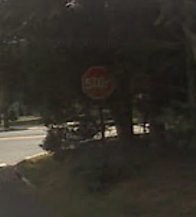In this small, dark image, the main subject is an awkwardly placed stop sign, located under a large tree. The stop sign is positioned off the street, on a small hill covered with yellow grass, green weeds, and possibly brown dirt due to the shading. Despite the tree's overhanging branches partly obscuring the sign, its octagonal shape and white letters spelling "STOP" are discernible. The background reveals a single-lane, bi-directional highway, although it's not directly aligned with the sign. Surrounding the area are several trees, creating a dense, dark backdrop that contrasts with the lighter foreground elements.